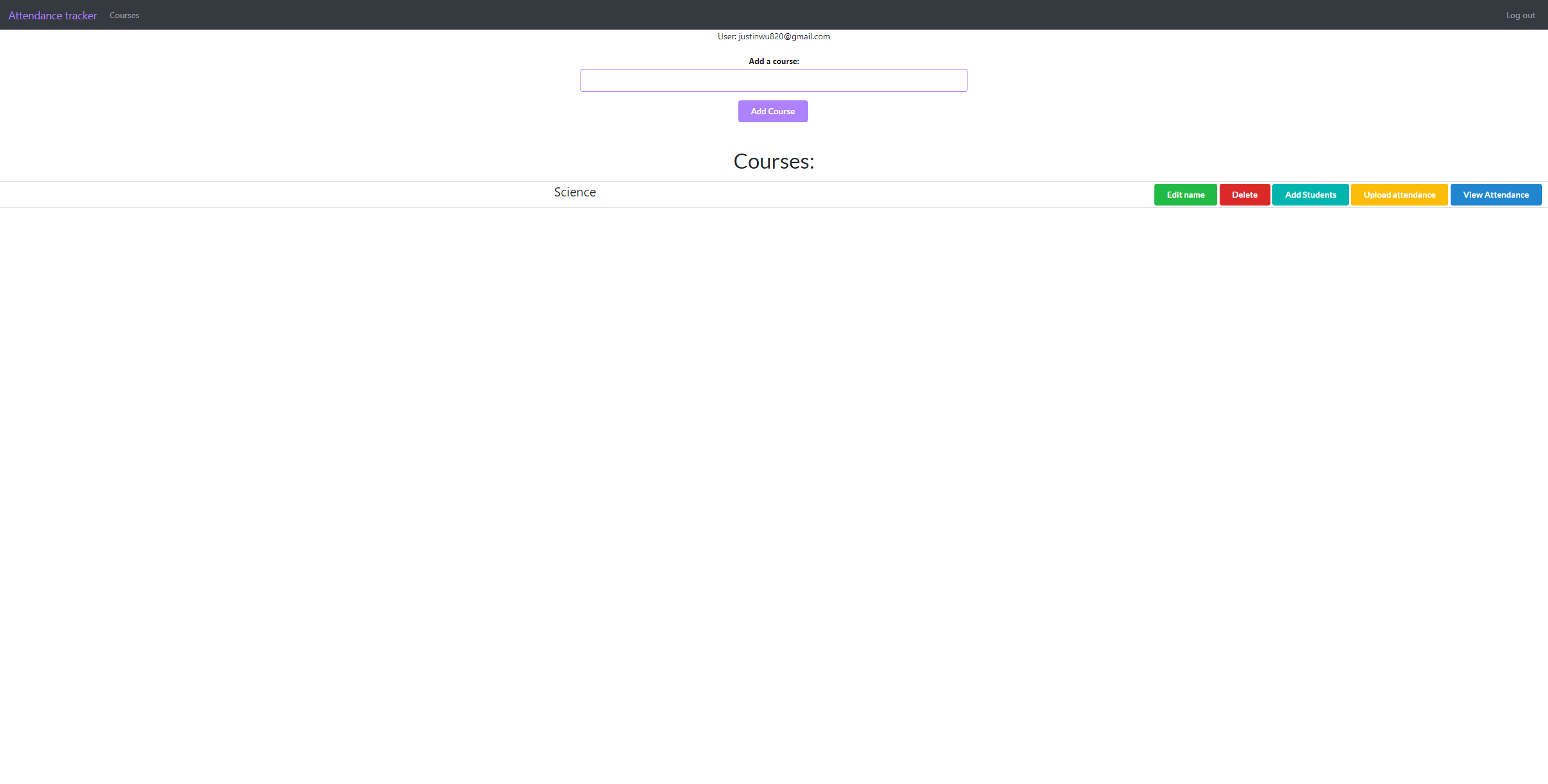The image appears to be a screenshot from an online course platform. At the very top, there is a black navigation bar with text on both the left and right sides, though the text is too small to discern. Below this, there is a header with some writing, followed by a search box. Underneath the search box is a prominent purple box with additional text inside. Below this, the section titled "Courses" is displayed, with "Science" labeled on the left. To the right of the "Science" label are five colored boxes organized in a row: green, red, aqua, yellow, and blue. The overall color scheme of the screenshot includes the black navigation bar, purple box, and the colorful boxes for course categories, against a primarily white background.